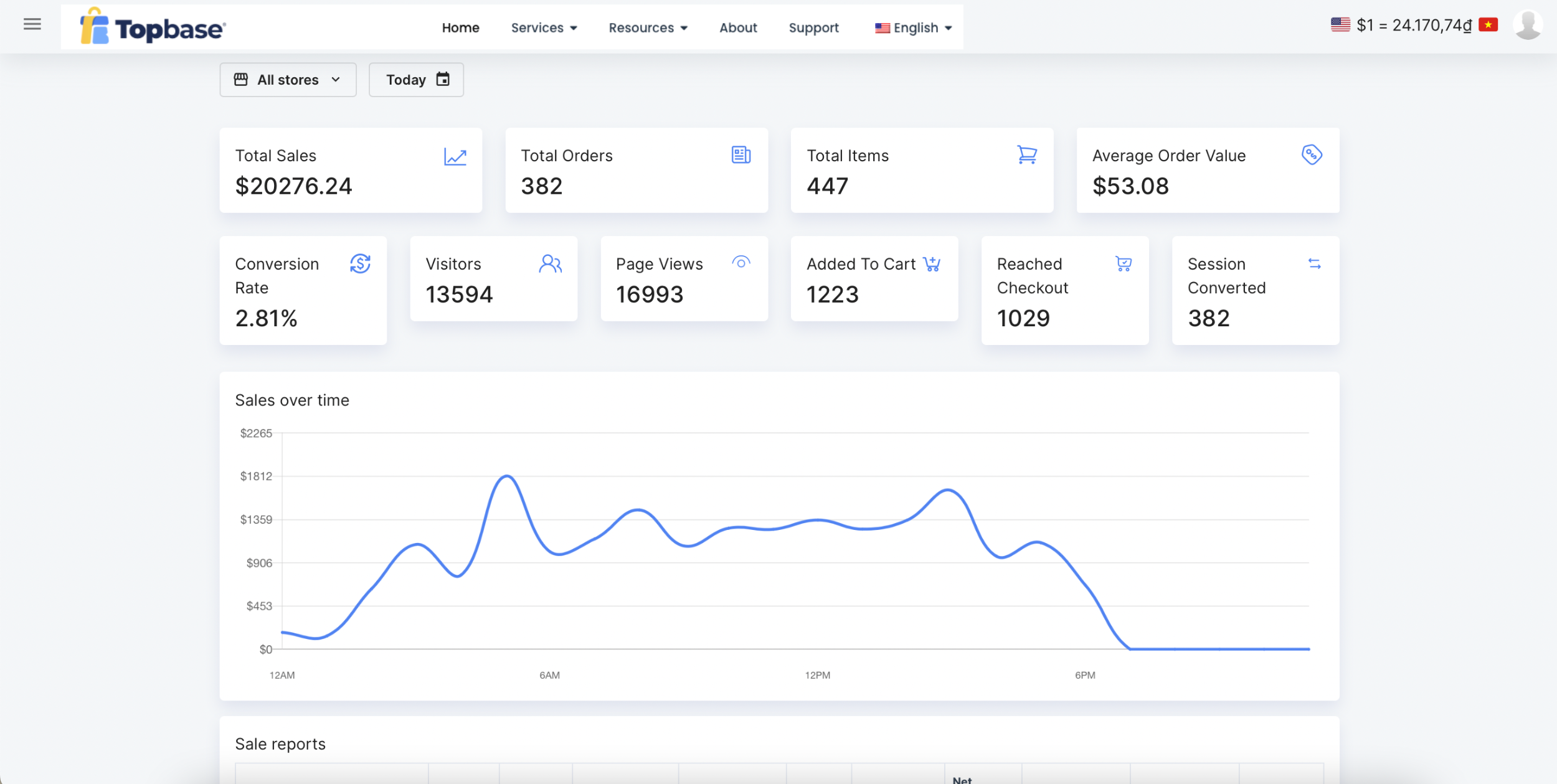**Caption:**

The image displays a stock market dashboard with a distinct layout. At the top, there is a bold heading that contrasts with the lighter subheadings. To the left of the "e" in the header is a floating registered trademark symbol, difficult to read. Adjacent to this, there is an icon resembling a blue present with a yellow ribbon, which is accompanied by three horizontal lines representing a settings menu.

The dashboard includes a navigation bar featuring options such as Home, Services with a drop-down menu, Resources, About, and Support. There's also a language selection option, currently set to English.

Displayed prominently is an exchange rate, showing one US dollar equals 24.17 units of another currency. Below this rate, there is a drop-down menu labeled "All Stores" which allows users to filter by specific stores, and a display of the current date which users can modify.

Further down, four key performance indicators are highlighted in separate boxes: 
1. Total Sales: $20,276.XX
2. Total Orders: 382
3. Total Items: 447
4. Average Order Value: $53.08

Following these metrics is another set of statistics, starting with the conversion rate at 2.81%, total visitors at 13,594, total page views at 16,993, items added to cart at 1,223, reached checkouts at 1,029, and sessions converted at 382.

At the bottom of the dashboard, there is a line graph illustrating sales over time. The y-axis ranges from 0 to 2,200, while the x-axis spans from 12 a.m. to 6 p.m. The graph shows fluctuating sales data represented with a blue line.